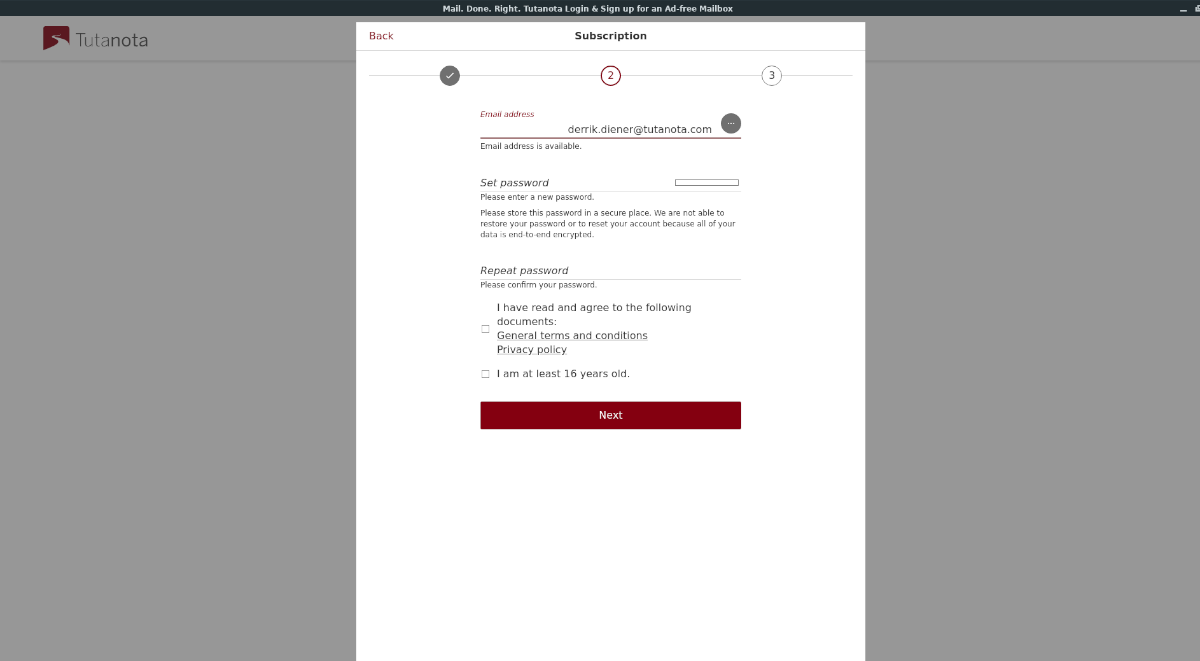This image depicts a webpage from Tutanota, a secure email service, prominently featuring a subscription sign-up form. 

At the very top of the webpage, there is a thin black banner that reads: "Mail Done Right - Tutanota." This banner includes options for users to login or sign up for an ad-free mailbox. 

Centrally located on the page is a white document form, flanked by dark gray borders on both the left and right sides. In the top left corner of the left gray sidebar, there is a distinctive red square icon with a white road winding up towards the word "Tutanota."

The primary document header is labeled "Subscription" in bold text. Just below this header, the word "Back" is highlighted in red. Below this, three horizontally-aligned circular progress indicators guide the user through the sign-up process. The first circle is dark gray with a white check mark, signifying completion. The second circle is outlined in red with a red number two inside, indicating the current step. The third circle is outlined in gray with the number three, representing the next step. A faint gray line connects all three circles.

Under the progress indicators, the label "Email Address" appears in red text. Below this is an input field containing an email address, accompanied by a dark gray circle with a white line through it, suggesting some form of status or icon. Following this entry field, a red divider line spans the width of the form. Beneath the line, on the left side, the phrase "Email address is available" is displayed.

Next in the form, the section labeled "Set Password" appears. To the right, there is an outlined rectangle designated for password entry. Underneath, a text prompt advises: "Please enter a new password." Further down, another prompt cautions users to "Please store this password in a secure place. We are not able to restore your password or reuse your account because all your data is end-to-end encrypted."

A small space below, the form asks users to "Repeat Password," followed by a thin dividing line and the instruction "Please confirm your password."

Towards the bottom of the form, users must check a small white square next to the statement: "I have read and agreed to the following documents," with "general terms and conditions" and "privacy policy" underlined for emphasis. Another small white square is next to the affirmation: "I am at least 16 years old."

Finally, at the bottom of the form, there is a large red rectangle with the word "Next" written in white, indicating the button to proceed to the next step of the sign-up process.